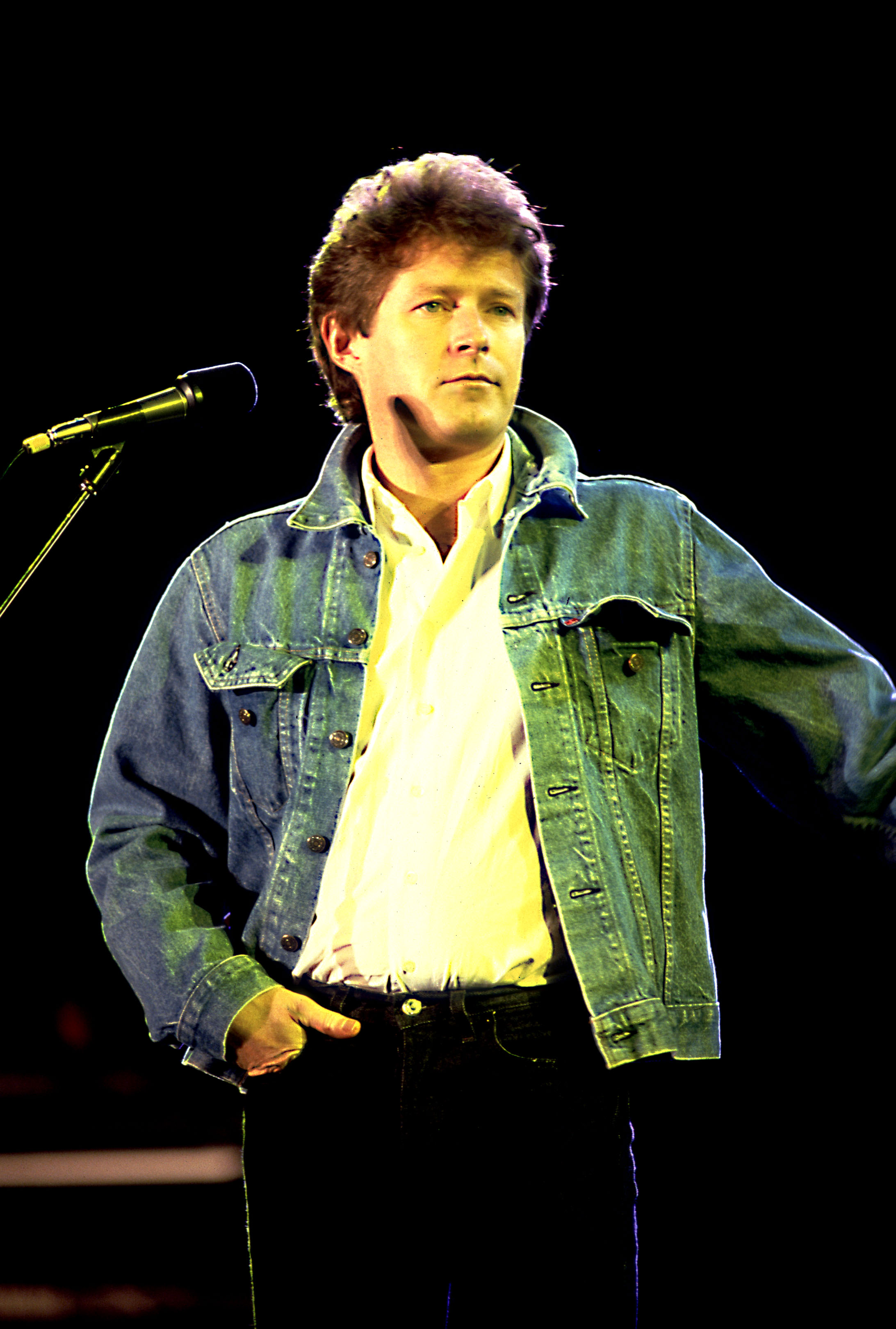In the image, you see a serious-looking white man standing on a stage with an all-black background. He has short brown, curly hair styled in an 80s mullet fashion. He is dressed in an unbuttoned denim jacket with a popped collar, over a collared white or yellow shirt, and black jeans with a visible gold button. The man has one hand in his pocket while the other is extended to his side. His gaze is directed slightly away from a microphone with a black fuzzy head positioned to his left. His facial expression suggests annoyance or reluctance, with furrowed eyes. Stage lights from behind illuminate the top of his hair, giving it a whitish glow, and cast a yellowish hue, enhancing the dramatic effect. At the lower left, there might be a white object such as a bar, handrail, table, or beam blending into the dark setting.